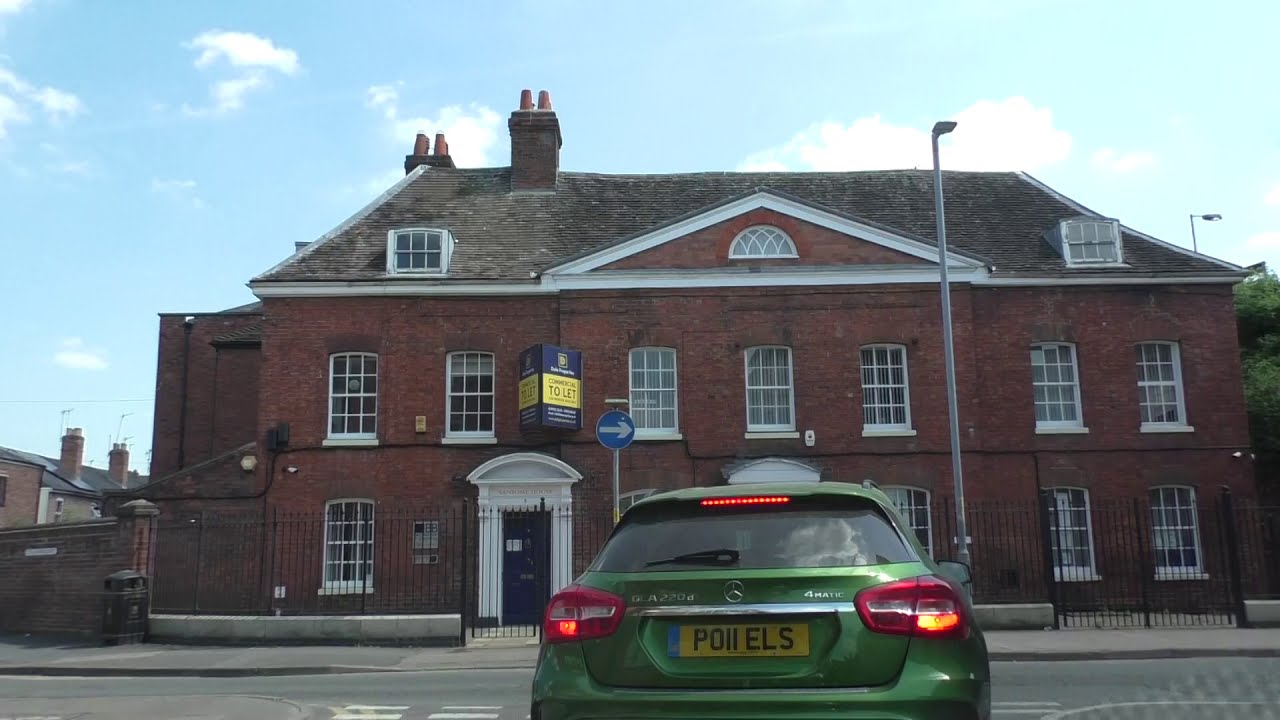The image showcases a large, aged red brick house resembling an old-school style structure, dominating approximately 70% of the background. The house is three storeys high, with the third storey integrated into the grey roof, which features white window dormers and two chimneys. The structure is adorned with numerous white-framed windows and features an entrance highlighted by white columns and black doors. Surrounding the property is an iron gate, mostly black, complementing the historic aesthetic of the building. Near the house, there's a prominent light pole and a blue street sign with a right-pointing arrow. 

In the foreground on a small portion of the road, a green Mercedes GLA-220D SUV with the designation "4MATIC" on the back is parked, showcasing red taillights, a small rear windshield wiper, and a distinctive license plate reading "P-O-I-I-E-L-S." The setting is bathed in natural daylight under a blue sky dotted with white clouds. Additional details include a yellow background sign with black text reading "Commercial 2LT," hinting at the building's potentially mixed usage. The amalgamation of these elements captures a scene typical of an architectural snapshot outside of the United States.